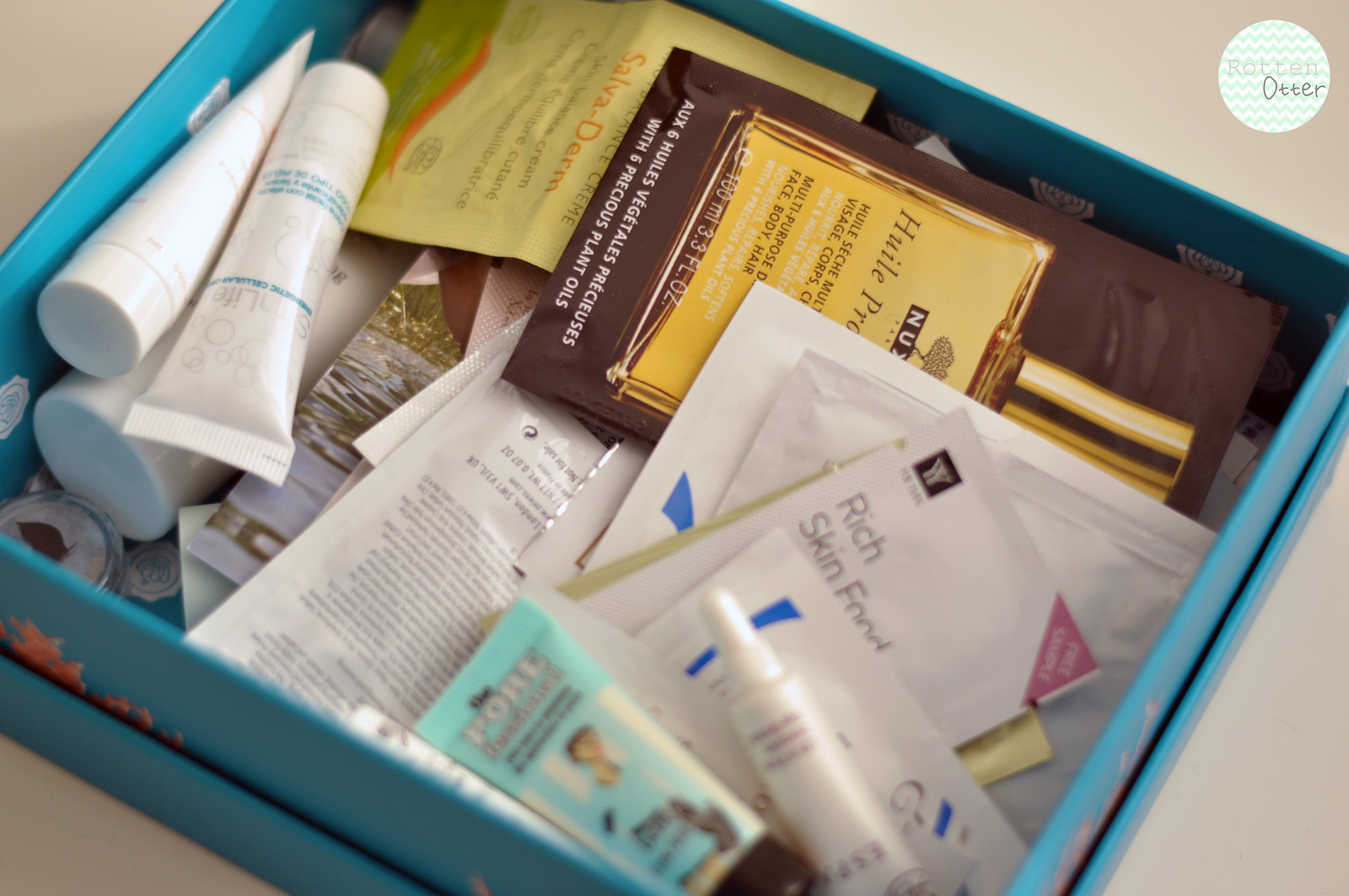This vibrant color photograph captures a blue box brimming with a variety of makeup and skincare samples, nestled within the box’s lid. Set against a beige background, the image is subtly branded by a logo situated in the upper right-hand corner, which features a white chevron pattern interlaced with green elements and the name "Rotten Otter." Inside the box lies an assortment of products: pouches, one noticeably labeled "Rich Skin Food," alongside several small tubes. Among these, a perfume sample is discernible, adding diversity to the collection. The contents, primarily skincare items in varying shades but predominantly white, are tightly packed, making it difficult to distinguish individual product names. The sample sizes suggest they are ideal for someone either looking to test various products or intending to use them for travel-friendly skincare and cosmetic needs.